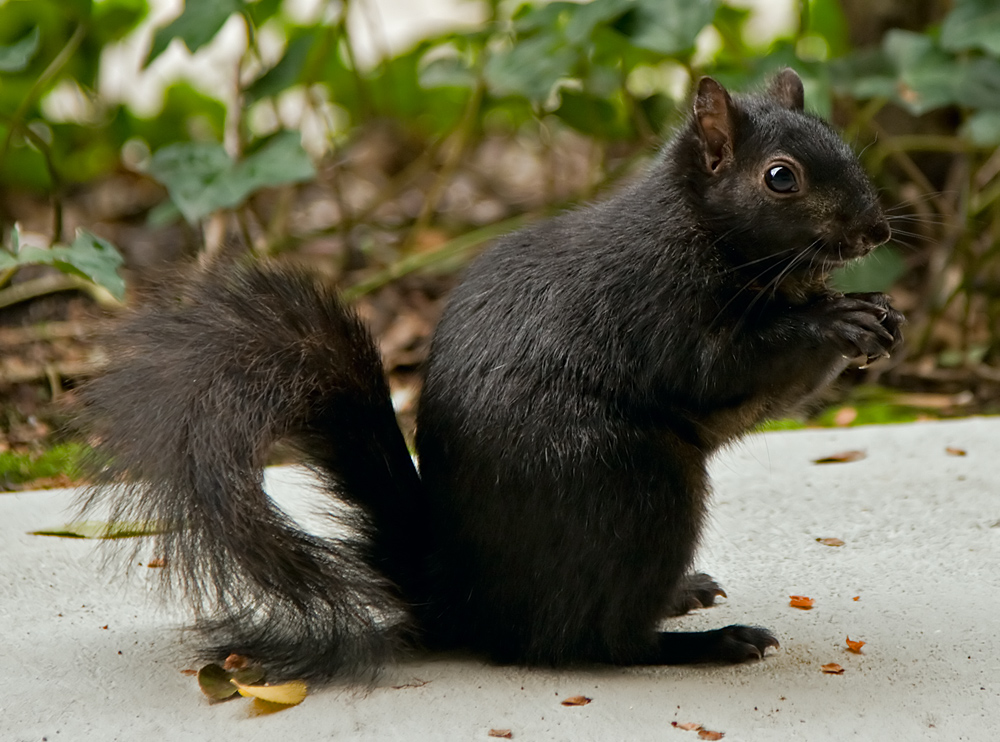The image depicts a very dark black squirrel, possibly dark brown, sitting upright on its haunches on a concrete surface resembling a human path. The squirrel's bushy tail is raised and curled under. Its face is in profile, revealing a large black eye, pointy nose, and rounded ears. The squirrel's front paws clutch a small object, likely a nut or piece of food, while its claws protrude from its bottom feet. The background is a blur of green foliage, plants, and shrubs, with several broken leaves scattered on the concrete around the squirrel. Its whiskers extend outward, adding to its cute and curious appearance.